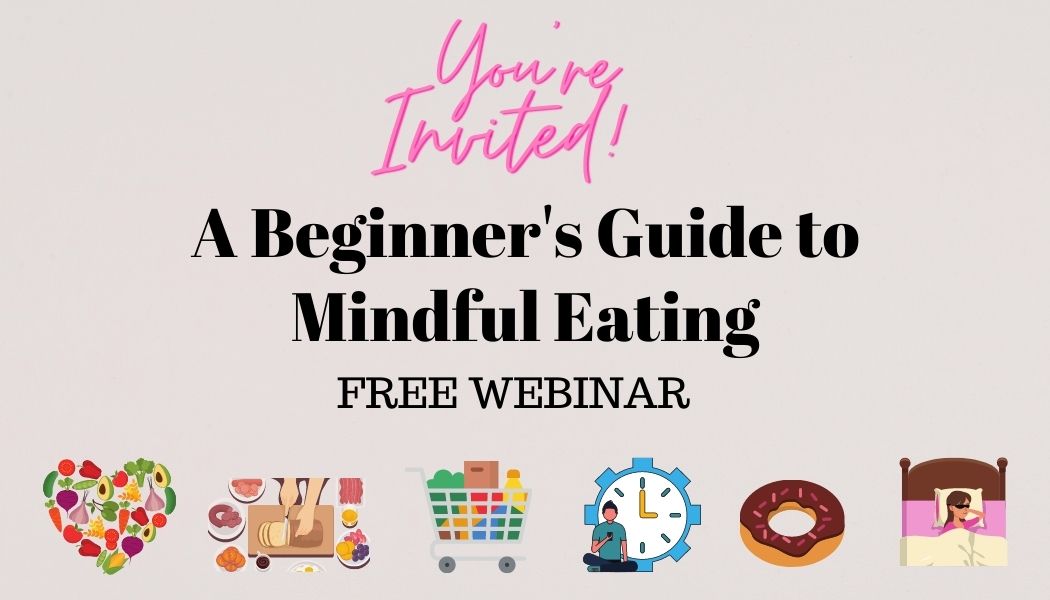Here we have an invitation featuring an elegant pink cursive script that reads "You're Invited!" against a rectangular, gray background. Below this, in bold black block lettering (not cursive), it says "A Beginner's Guide to Mindful Eating." Under that, in plain black uppercase lettering, "FREE WEBINAR" is prominently displayed.

The invitation is visually engaging with several colorful and cartoonish graphical icons:

1. A heart composed of vibrant fruits and vegetables.
2. A person cartoonishly cutting bread on a cutting board, surrounded by various types of food including vegetables and meats.
3. A grocery cart brimming with an assortment of groceries, including green leafy vegetables.
4. A person meditating in front of an oversized clock, perhaps a stopwatch.
5. A mouth-watering donut with chocolate icing and sprinkles.
6. A woman in bed wearing an eye mask, nestled under white sheets and a brown wooden headboard, lying on pink sheets with a white blanket.

The visual elements make the invitation lively and informative, with each icon symbolizing different aspects of mindful eating and related lifestyle choices.